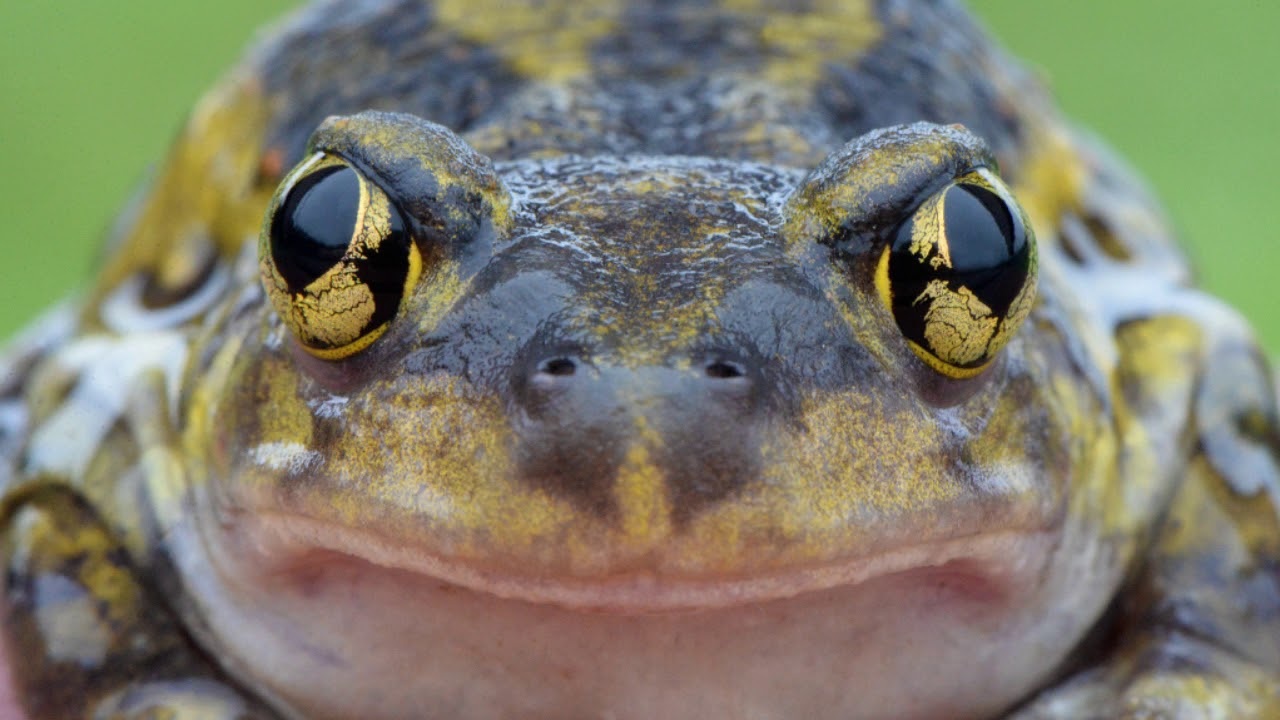This highly detailed, ultra close-up color photograph captures a frog looking directly at the camera, which appears to be mere inches from its face. The frog occupies almost the entire frame, with only the corners showing an out-of-focus, medium green background, suggesting it is outdoors, possibly on grass. The frog's face is sharply in focus, while its body, shoulders, and upper legs are slightly out of focus.

The frog’s skin is predominantly dark grayish-black with vibrant yellow stripes and speckles. Its prominent nostrils are positioned centrally on its snout. The frog’s eyes are dramatic, with deep black pupils surrounded by golden-yellow irises, featuring black splotches and thick, rubbery-looking eyelids that bulge outward.

Its mouth, which extends horizontally along the bottom of the photo, is a pinkish-peach color and closed, giving the appearance of a slight smile. The frog's upper lip has a yellowish hue, and the area beneath the mouth is white. Despite its blurred body, the intricate pattern of its dark and yellow-striped skin is evident. This image offers an intimate and high-quality view, making the viewer feel as if they are face-to-face with the frog, gazing into its eyes.